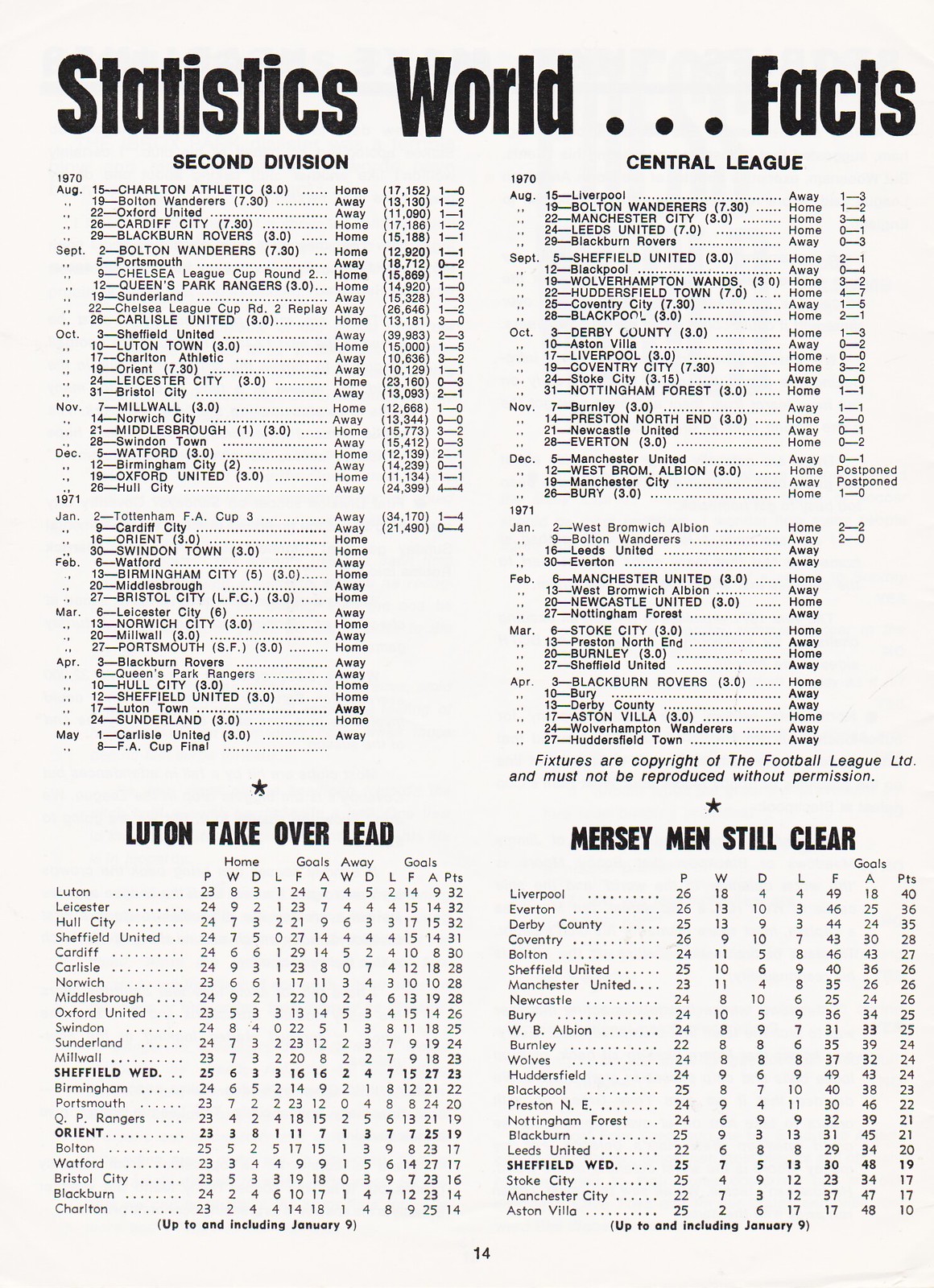The black-and-white image depicts a historical soccer statistics sheet with a creamy, aged-white background. Dominating the top of the page in bold black letters are the words "Statistics World... Facts." The sheet is divided into four sections, with the top labeled "Second Division," featuring detailed records of soccer clubs' games from August 15, 1970, through May 1971. Clubs such as Sheffield United, Luton Town, Charlton Athletic, Bristol City, Watford, Birmingham City, and Oxford United are listed, along with their game dates, outcomes, home or away statuses, and scores, although some entries are awaiting details for yet-to-be-played matches. Below this section, the sheet is horizontally bisected into two more sections. On the left, the heading reads "Luton Takes Over Lead," while on the right, "Mercy Men Still Clear" governs the information. A small black star is nestled between these two lower columns, bridging the detailed chronicles of soccer prowess.